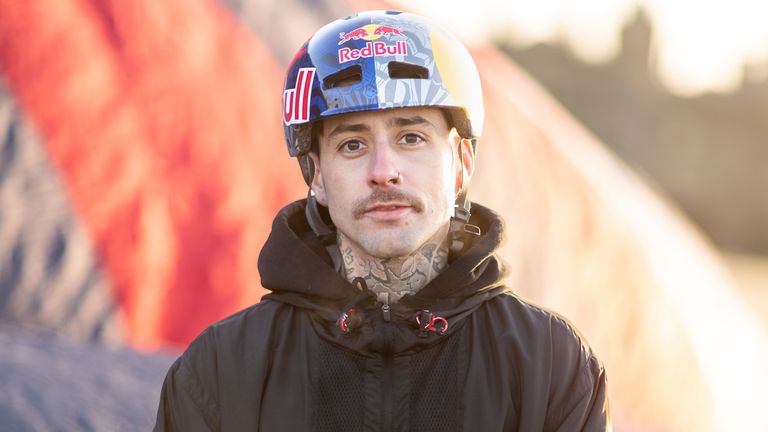A close-up image captures a man staring directly into the camera with an intense gaze. The photograph is tightly framed, cutting off just below his shoulders and mid-chest, ensuring his face and upper torso dominate roughly 60% of the image. He wears a distinctive protective half-helmet, which provides no facial coverage, revealing his determined expression clearly. The helmet sports a gradient design, transitioning from a dark blue on the left side (his right shoulder) to a lighter blue on the right, prominently featuring a Red Bull sticker. The background of the image is bathed in a striking play of colors, with hues of purple and reddish tones enveloping the left side of the frame, accentuating the man's right shoulder, creating a vivid and dynamic contrast that highlights the subject.